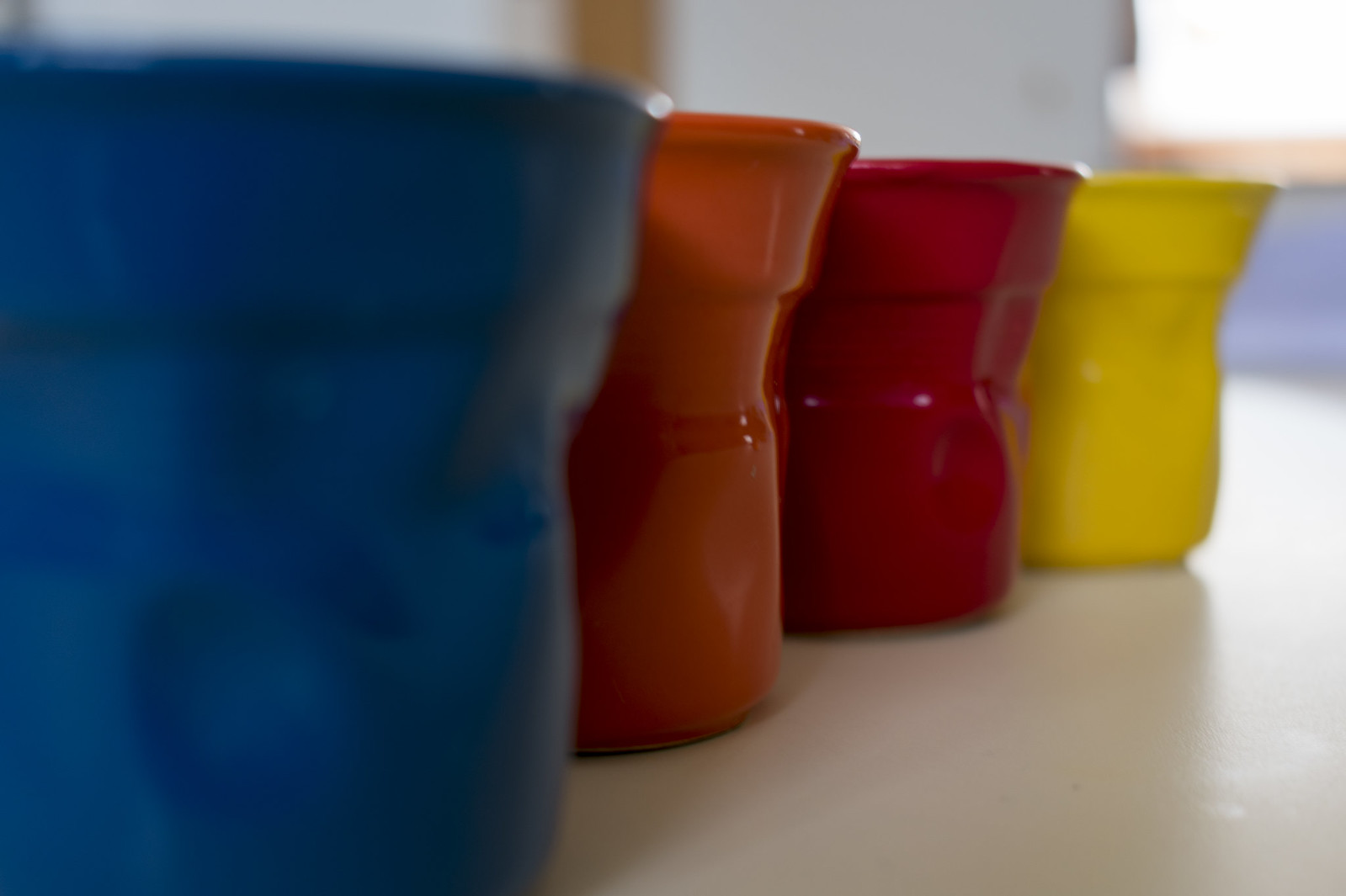The photograph captures four ceramic containers, all of the same shape but in different colors: blue, orange, red, and yellow, arranged on a white surface in an indoor setting. The blue container, positioned closest to the camera on the left, is the largest and most blurred, with the blurriness extending to the table and the general background. The orange and red containers, located in the middle, are clearer and more defined. The yellow container, situated farthest from the camera, is also somewhat blurred but not as much as the blue one. Sunlight appears to be streaming in from outside, casting shadows and adding a touch of blue to the distant blurred wall. The entire picture has a rectangular composition, offering a side view of the containers.